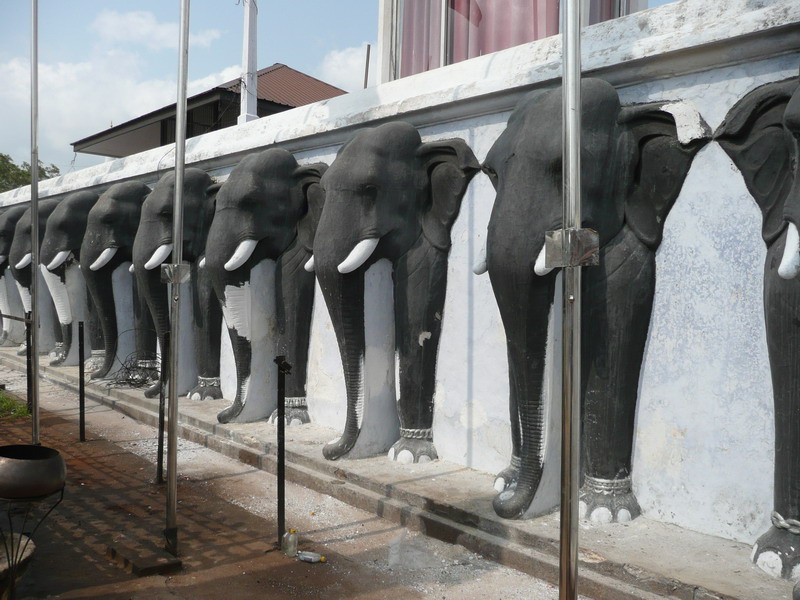The image depicts a long white concrete wall, approximately 12 feet high, adorned with several large, detailed elephant statues. These statues, appearing as if they are emerging from the wall, display only the front parts of the elephants, including the head, large ears, tusks, trunks reaching down to the sidewalk, and the front legs with silver feet and white toes. The tusks are predominantly white with some gray elements, possibly for support. The elephants are positioned in a row along the entire length of the wall, some showing signs of wear and chipping. In front of the wall, there is a deteriorating brick structure featuring supports, remnants of an old railing, and a tin container on wrought iron stands. Behind the wall, a pink and white structure and a building with a brown roof are visible in the background. The scene includes a sense of disintegration with some debris apparent near the elephants' feet.